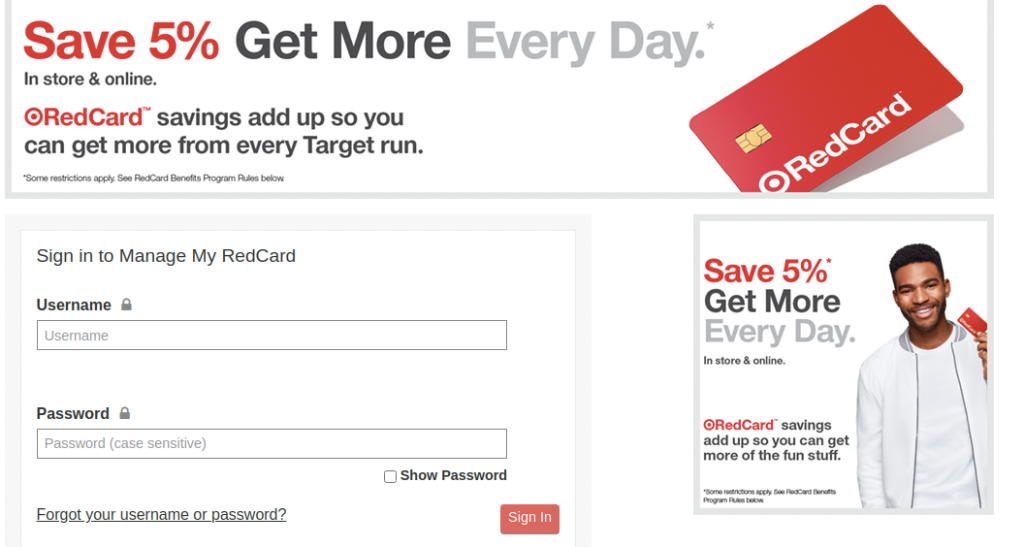The image is a wide rectangular banner with a predominantly white background. At the top of the banner, large red text reads "Save 5%," with the phrase "Get More" in smaller black font to its right, and "Everyday" in gray font further to the right. Directly below the "Save 5%" text, aligned to the left, smaller black text states "in store and online."

Beneath this section, there is the Target logo in red followed by the text "REDcard™" also in red. Below that, in black, the text reads "Savings add up so you can get more from every Target run." To the right of this text, there is an image of a REDcard; the card is red with the Target logo on the left and the word "REDcard" in white, featuring a gold chip typically used for scanning.

In the section below, on the left-hand side, the text "Sign in to manage my REDcard" appears. Under this, there is a label "Username" next to a lock icon, with a blank input field below it that displays "Username" in light gray text as placeholder text. Next, the label "Password" appears next to another lock icon, with a blank input field below stating "Password (case sensitive)" in light gray text.

Towards the lower right of this section, there is a checkbox with the label "Show password." Finally, at the bottom center of the page, a prominent red button reads "Sign in."